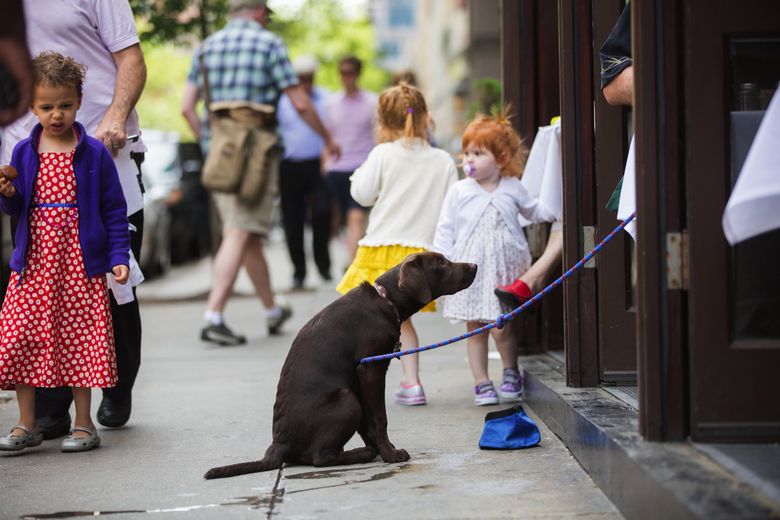This detailed photograph captures a bustling street scene with its primary focus on the sidewalk. Center stage is a brown Labrador seated on the concrete, attached to a purple and red striped rope leash. The leash is connected to a table in the open patio area of what appears to be a restaurant; the fringes of tablecloths are just visible through the open doors leading out to the sidewalk.

Surrounding the dog are three young girls. On the left, a girl with dark curly hair, wearing a red and white polka dot dress under a purple fleece jacket, stands holding an older person’s hand. She’s wearing gray Croc-like sandals and looking down with a scrunched-up, slightly upset face. 

In the middle of the photo, a girl with her back turned to the camera wears a cream-colored sweater over a yellow skirt. To her right is a younger girl, possibly her sister, wearing a white dress and sweater, with striking red hair and a pacifier in her mouth. She also has on purple shoes and appears to be blowing a bubble.

In front of this little girl is the dog on the leash, looking intently toward the table it’s tied to. A blue bag is placed in front of the dog. 

In the background, several adults are visible, though they appear out of focus. A person in a lilac-colored shirt stands behind the girl with dark curly hair, while a man in a plaid short-sleeved shirt and khakis walks away, carrying a bag over his shoulder. Two other men, one in a pink shirt and another in a blue shirt, are walking toward the camera.

The scene is lively, filled with interactions and captures the everyday moments that compose a street-side atmosphere.